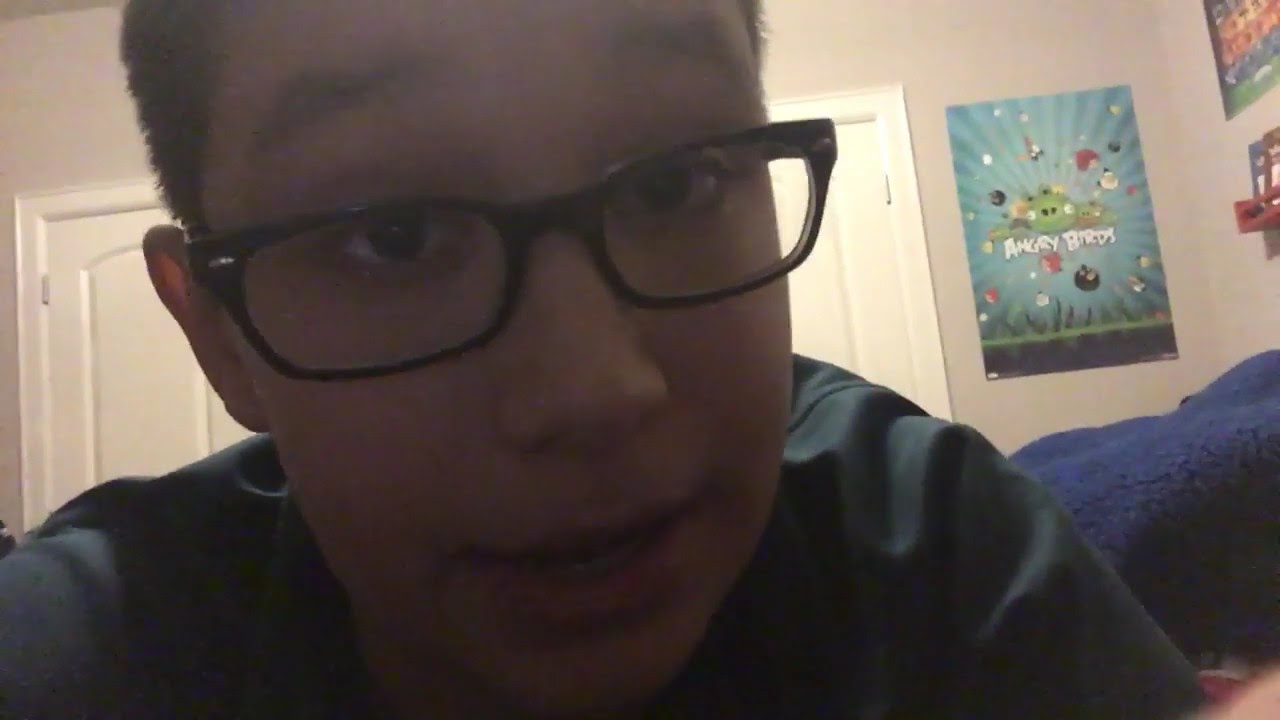This image depicts a young boy, likely in his early teens, with a buzz cut of very short dark brown hair and brown eyes. He wears heavy-framed, square-shaped black glasses and a dark green t-shirt. The boy is looking directly into the camera, speaking with his mouth open, displaying his lower row of teeth, suggesting he might be in a video chat or recording himself. The focus is prominently on his oval-shaped face with noticeable cheeks, obscuring much of the background. Behind him, his bedroom features light tan walls, two white doors, and a blue-covered bed. The most striking elements are the posters on the walls, particularly an Angry Birds poster with a blue background and the prominent green pig character at the center.